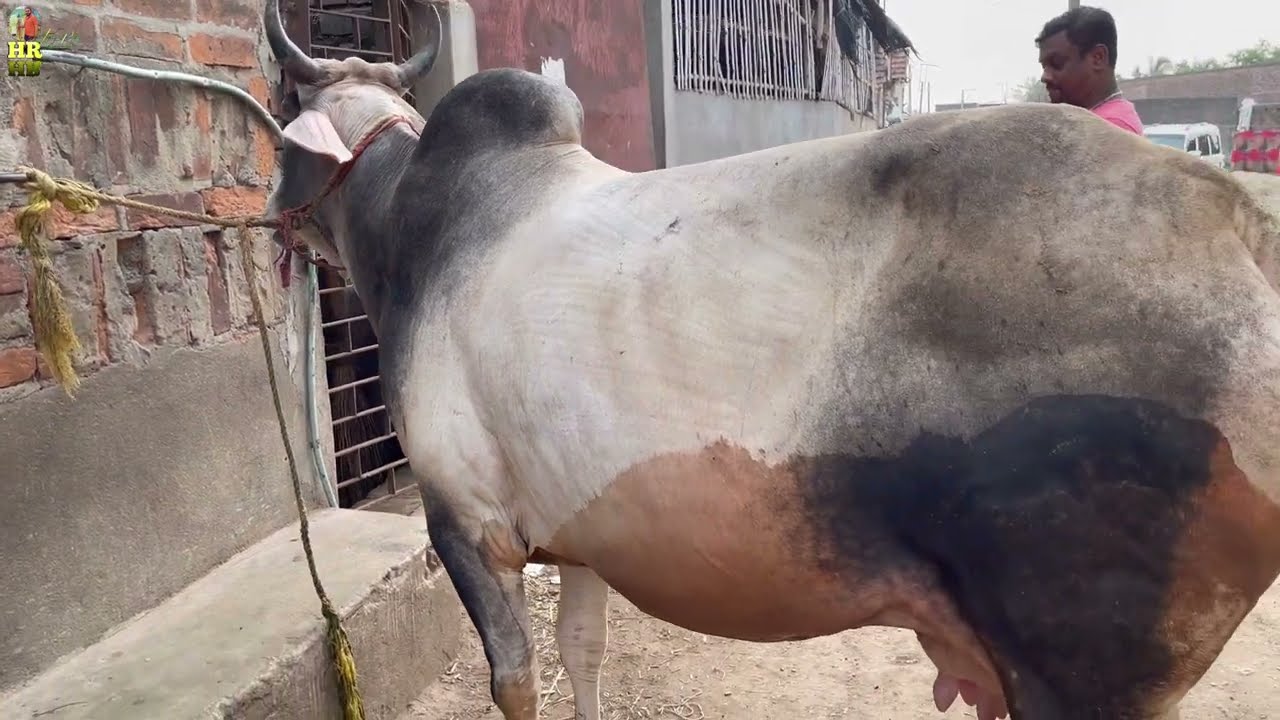In this detailed street scene, likely set in a country like India, we see a side view of a cow, which might be mistaken for a bull or a water buffalo due to its mixed colors and features. The cow is tethered with a rope to an old brick and concrete wall that's situated along the left side of the street. The cow has a distinctive fur pattern: its middle section is white, while the front and back parts are black, with some tan and gray patches, giving it a somewhat dirty appearance. It also has a single hump and horns. There's a metal door with cutouts embedded in the wall and a concrete bench nearby. The background shows rundown buildings, including a torn window, adding to the rustic atmosphere. Behind the cow stands a man, partly visible, with tan skin and short dark hair. He is wearing a bright pink T-shirt, adding a pop of color to the scene. The lighting suggests an overcast sky with light gray clouds, casting a diffused light over the entire location. Two ropes are attached to the cow: a red one around its head and another yellow one hanging down toward the ground.